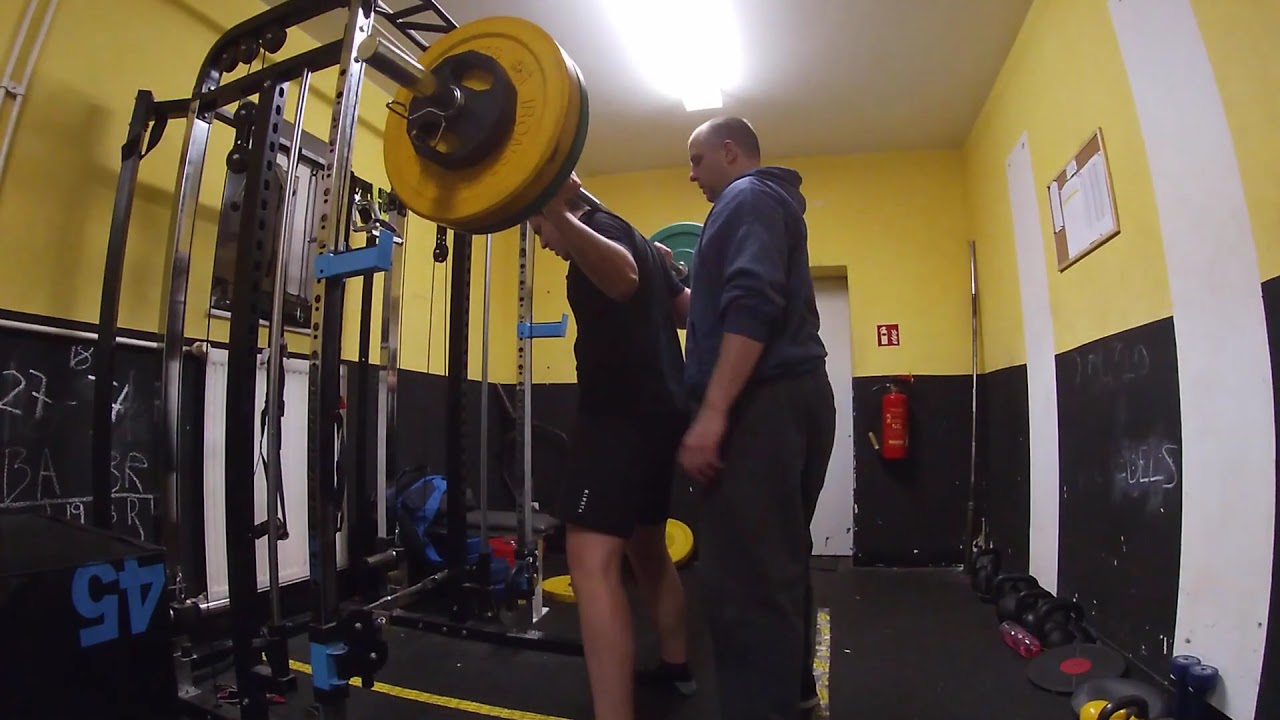This horizontally aligned rectangular photograph captures a scene inside a narrow weight room in a gym, characterized by its yellow upper walls and chalkboard-like black lower walls with some white writing on them. The ceiling is white, featuring a partly visible fluorescent light. The floor is black with various weights, including dumbbells, lying around.

At the center of the image, a man with a short-sleeved black t-shirt and black shorts is performing a squat while holding a barbell with large, colorful weight plates—yellow on the left and green on the right—positioned behind his neck. His side profile suggests he is Caucasian, though it's not entirely clear. Close behind him, a bald or nearly bald older man with very short brown hair, wearing a navy blue hoodie with the sleeves pushed up and black pants, is spotting him.

Additional details include a small "EXIT" sign and a fire extinguisher on the far wall, a visible door, a rack with weights on the right, and an upside-down number "45" written on the left wall. Both men's attentive postures and the significant amount of weight being lifted lend a sense of intensity and focus to the scene.